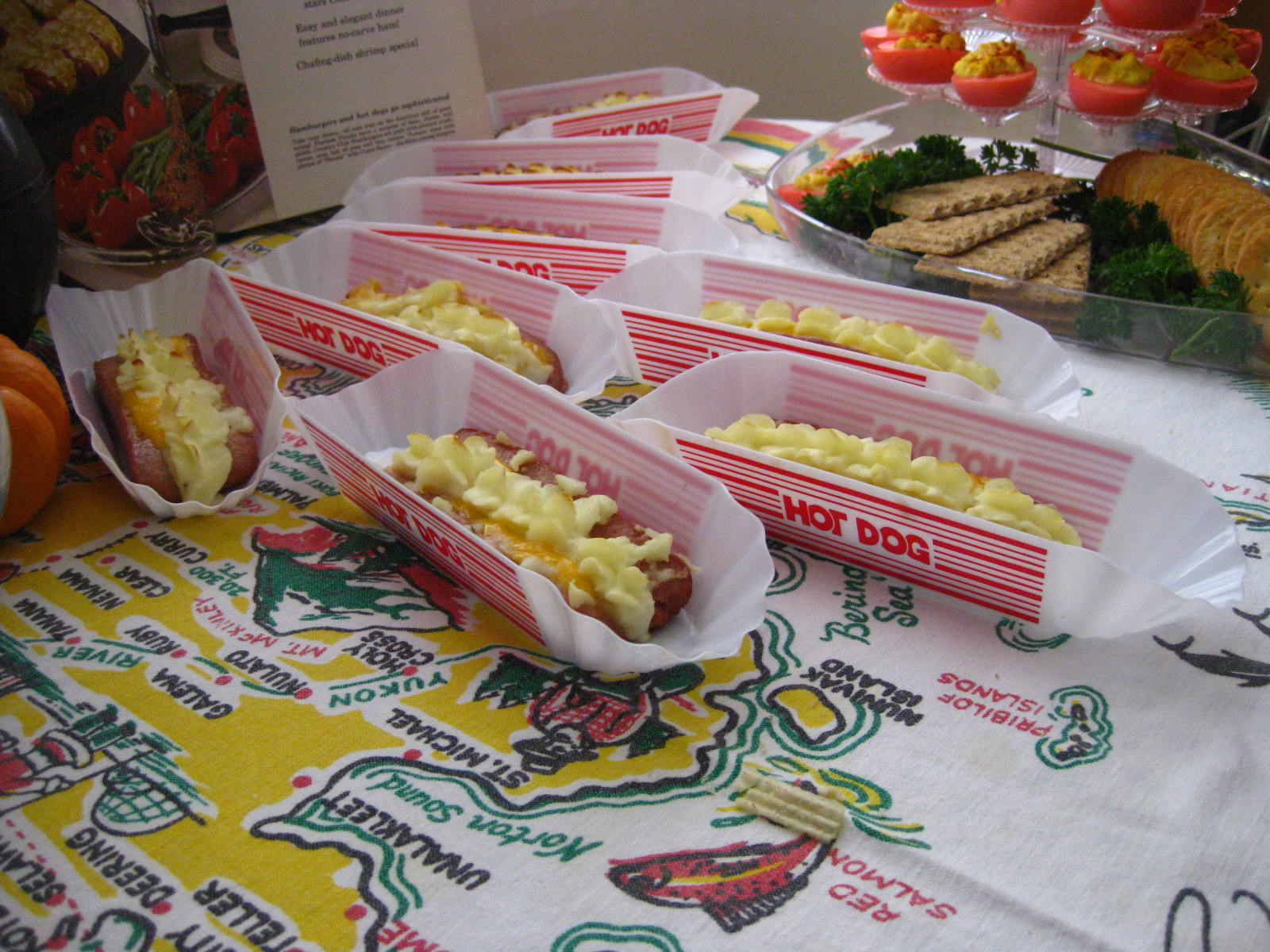This indoor photograph captures a party spread set on a table adorned with a vibrant tablecloth that features a detailed map. The map's yellow landmasses are decorated with city names in black text, marked by red dots, and include charming illustrations such as pine trees, a lumberjack resembling Paul Bunyan, green mountains, an igloo, and a Santa Claus figure. A prominent red salmon leaps from the map's depicted ocean.

On the table, there are approximately eight little white trays lined with red stripes, each labeled "hot dog" in red text. Each tray appears to contain a hot dog, though the exact contents are somewhat obscured by a fluffy yellow substance, which could be cheese, eggs, or a creamy topping.

To the back of the table is a tiered plastic food display. The bottom tier is garnished with green parsley and hosts an assortment of brown and rectangular crackers. Above it, the second tier features what seem to be pink deviled eggs, their halved, red-tinted shells cradling a yellow filling. To the left, there are some oranges, and an open cookbook displaying roasted red bell peppers, suggesting additional culinary inspirations for the event.